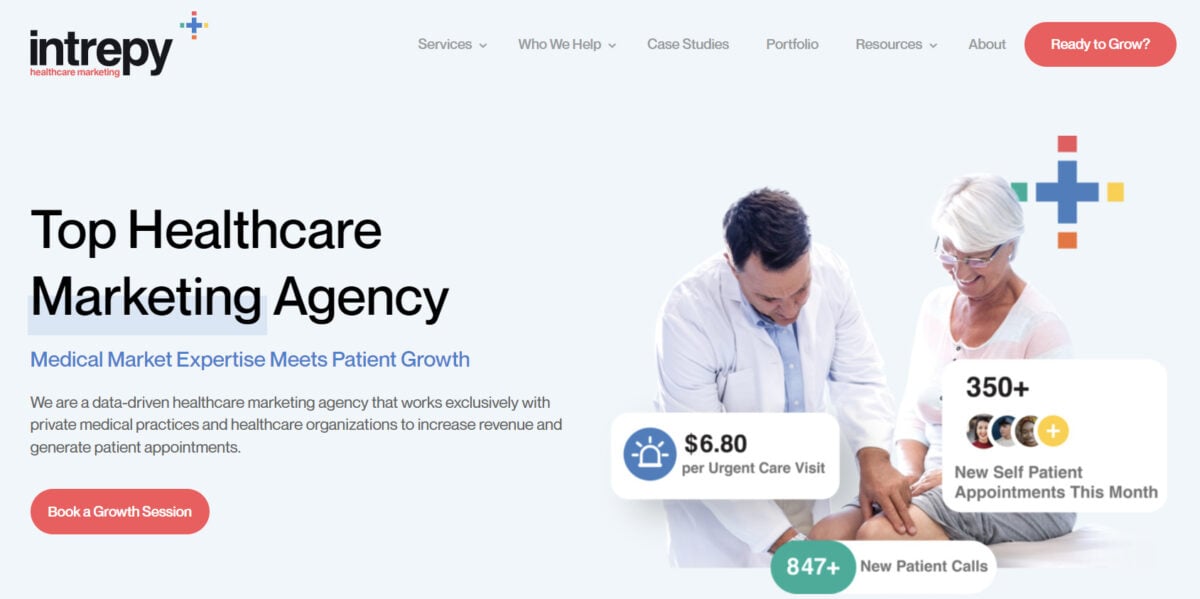The image depicts a website with a light gray background. At the top, the website's name, "Intrepy," is prominently displayed in bold black lowercase letters. Below the name, "Healthcare Marketing" is printed in red. 

On the right side of the header, there are several drop-down menu options: "Services," "Who We Help," "Case Studies," "Portfolio," "Resources," and "About." A red button labeled "Ready to Grow?" in white text is also situated on the right side.

Moving further down, on the left side, the text "Top Healthcare Marketing Agency" is visible. Beneath this, in blue print, it reads "Medical Market Expertise Meets Patient Growth." A brief paragraph follows this statement, accompanied by a red background button with white text that says "Book a Growth Session."

An image of a doctor and a patient is displayed, along with statistics in white text against a red background: "$6.80 per urgent care visit," "$350+ new self-patient appointments this month," and "$847+ new patient calls." There is also an icon of a head with a plus sign next to it.